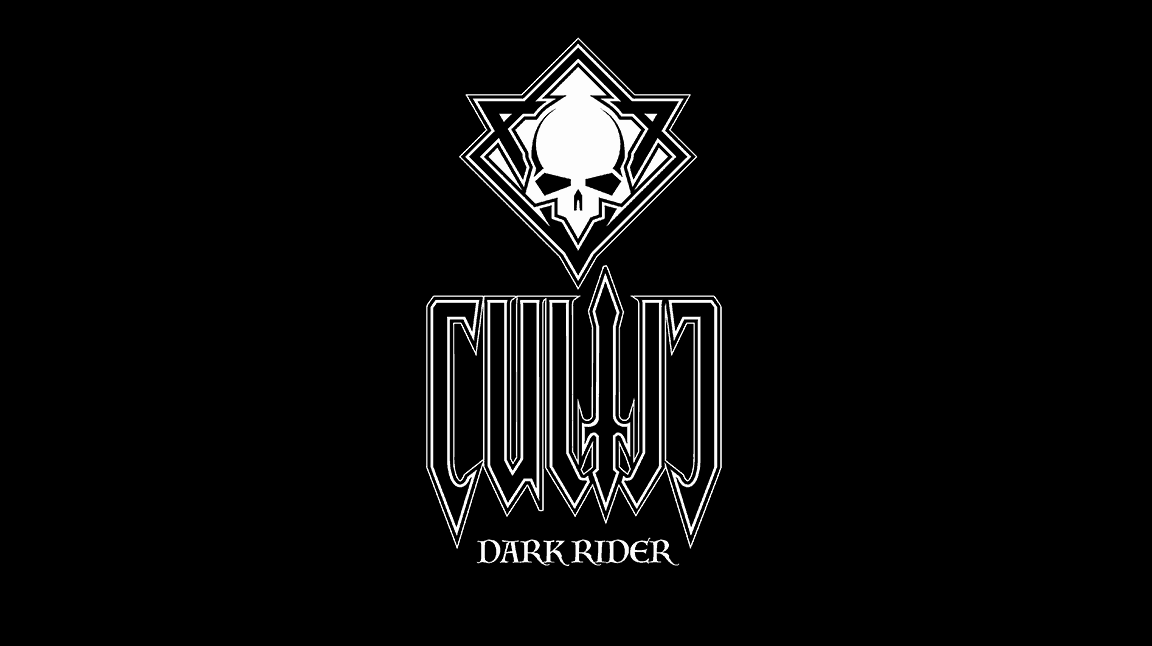The image features a large, horizontal black rectangle as its background. Centrally positioned, there is a series of layered white shapes and figures. At the top of this central design is a white diamond shape, outlined with alternating thin black and white borders. Inside the diamond, there is an inverted white triangle overlapping with the bottom half of a white skull, creating a distinct layered effect. Beneath these shapes, a series of intricately close-knit letters spell out "CULT" followed by a mirrored "LC," with a sword-like "T" featuring a diamond hilt amidst the letters. At the very bottom, in bold white font, are the words "Dark Rider."